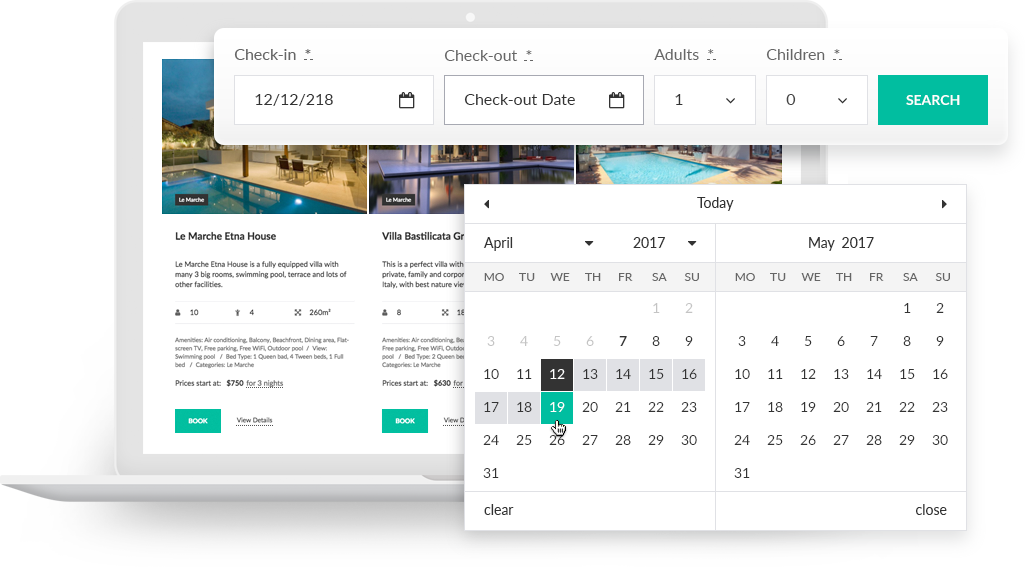A detailed photo collage captures a distinct juxtaposition of elements centered around an online hotel booking process. In the background, there's an image of a sleek white computer. Overlaying this image is a hotel search box interface, a familiar sight on many booking websites. This interface prominently displays four essential options: a section to input the check-in date, the checkout date, the number of adults, and the number of children. The interface, predominantly white with text in various shades of black, stands out crisply against the backdrop.

Particularly eye-catching is the vibrant green rectangle that serves as the "Search" button; inside the button, the word "search" is printed in a clean white font. Adjacent to the search box is a calendar interface, highlighted to show the selected dates for check-in and checkout. However, a noticeable error is present: the check-in date is listed as "12-12" and the checkout date is mistakenly entered as "2-18" instead of "20-18." This date discrepancy has caused a miscalculation, prompting the calendar to display dates from April 2017, thus disrupting the booking process and illustrating the importance of correct date entries in the user interface.